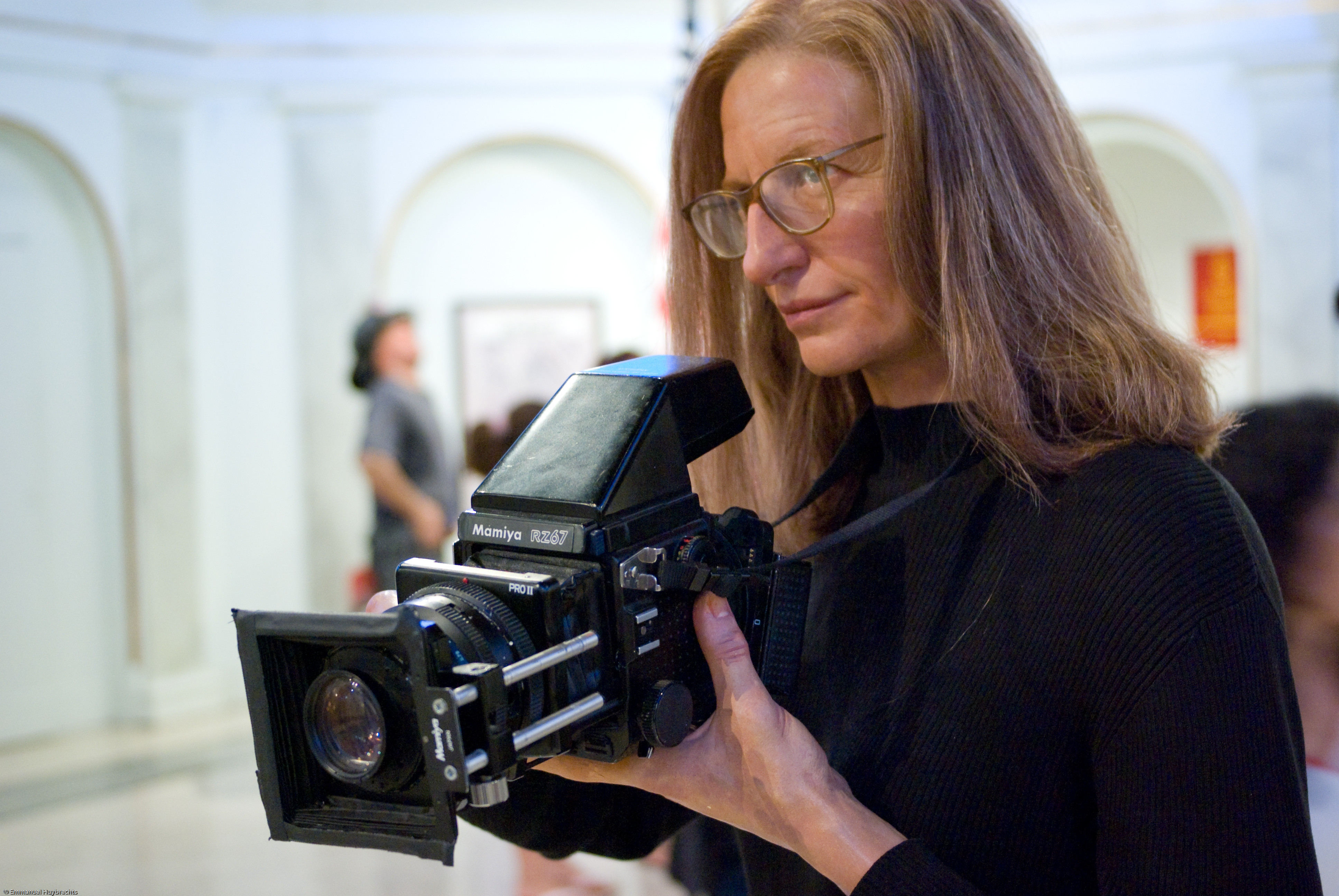The photograph captures a professionally-dressed woman holding a high-end Mamiya RZ67 Pro II camera. She sports a tall-collared, long-sleeve black shirt with a ribbed texture, paired with brown-rimmed glasses that frame her face. Her long blonde hair flows down to her shoulders and is parted in the middle. The woman, who appears to be older with some wrinkles around her eyes and forehead, has blue or green eyes and stands focused, directing her attention toward the left side of the image. In the background, a mostly white, possibly museum setting with indented arches containing paintings can be seen. The room's reflective white marble or tiled floor adds to the clean, crisp environment. A second person, wearing a hat and also looking upwards, is faintly visible behind her.